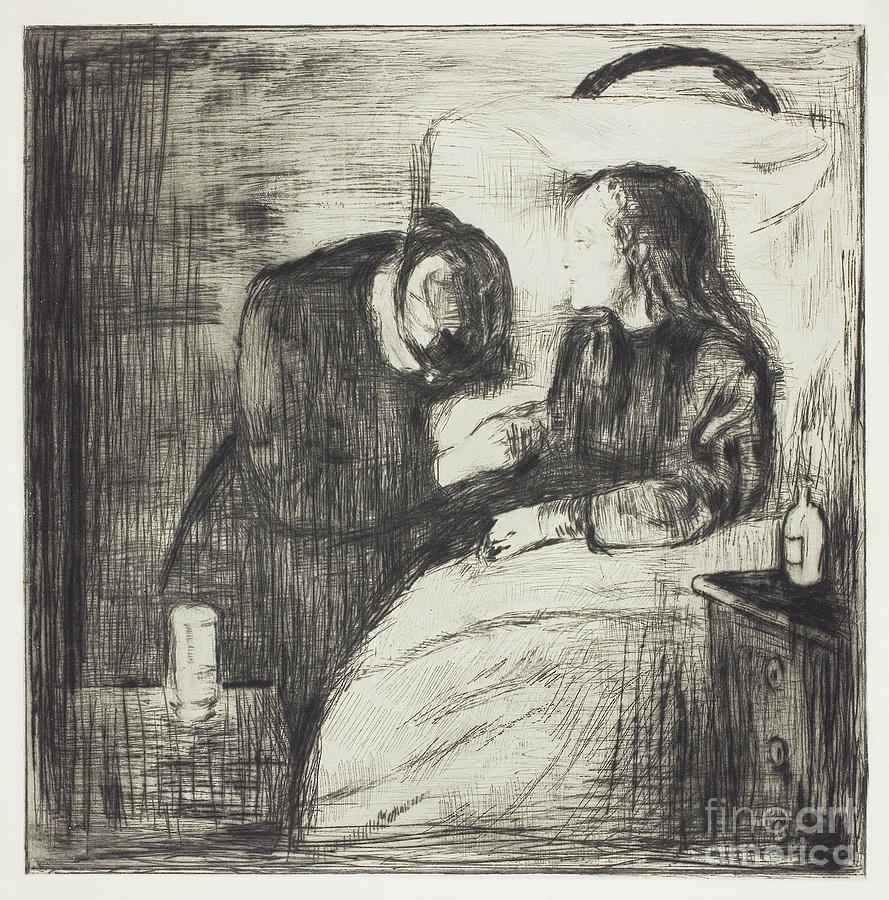This black and white pencil drawing, potentially crafted with charcoal or graphite, portrays a deeply emotional scene with intricate details. On the left side of the image, a person, whose gender is indistinguishable, appears to be kneeling or crouched down with their head bowed and dressed in dark clothing, giving an air of sadness or contemplation. To the right, a female figure sits in a chair with her long, dark hair cascading down and her eyes seemingly closed in somber reflection. She rests her arm across a blanket covering her legs and wears a long-sleeved top. Directly beside her, a small table holds a bottle, while towards the bottom left, a candle can be faintly discerned. The piece skillfully utilizes different shades of black, gray, and off-white to depict the features and elements within this indoor setting, creating a powerful contrast and depth in the artwork. At the bottom right, the drawing is signed with the phrase "Fine Art America."